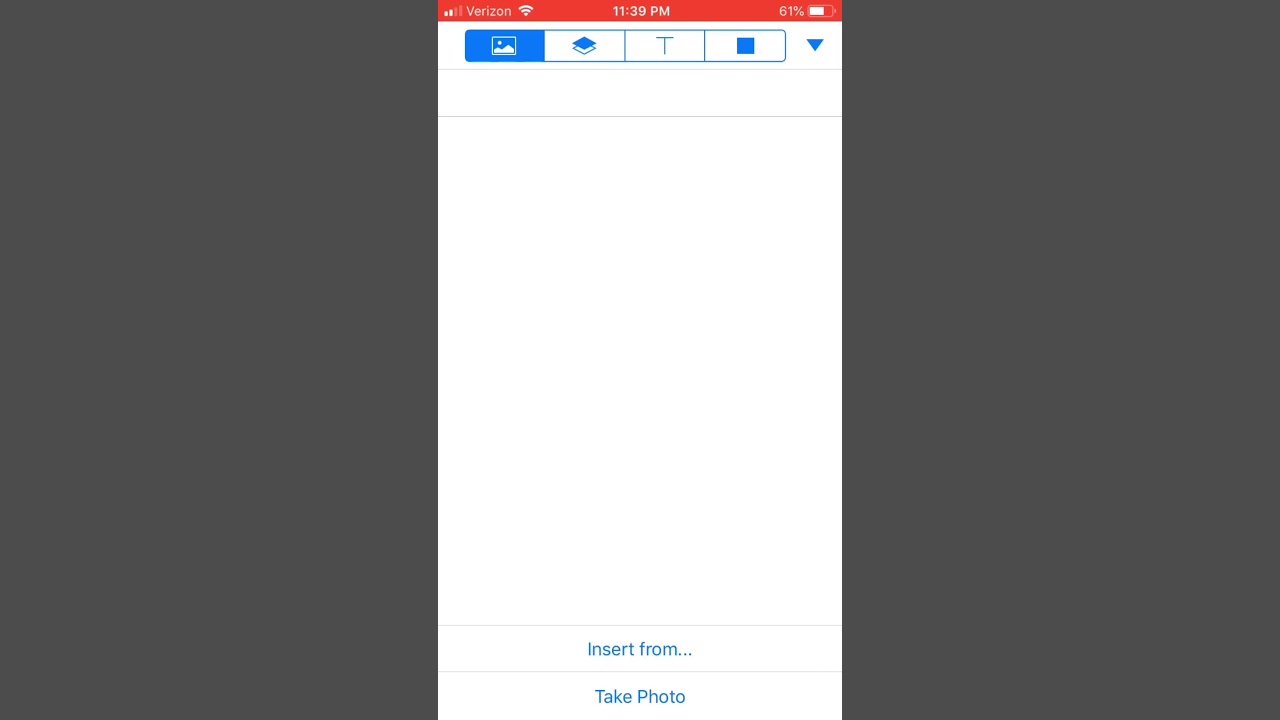The image is a horizontally oriented rectangle with a dark gray background spanning the entire width. Centrally positioned within this dark gray background is a vertical white rectangle. At the very top of the image, there's a red bar followed by a white section displaying system information: "Verizon," a Wi-Fi connection indicator, the time "11:39 PM," and a battery level at "61%."

Below this information section, a vertically centered white rectangle contains various logos. The highlighted logo in blue appears to depict a landscape photograph. Adjacent to this, on the right, is a blue square stacked on a white square, followed by a capital "T." Continuing to the right, there's another blue square, this time accompanied by a blue downward-facing arrow, signifying a dropdown menu.

Further down, two pale gray lines segment the white rectangle, creating a large expanse of white space. Below this white space, another pale gray line is followed by text in blue that reads "Insert from...". Another pale gray line is present below this, with blue text stating "Take photo."